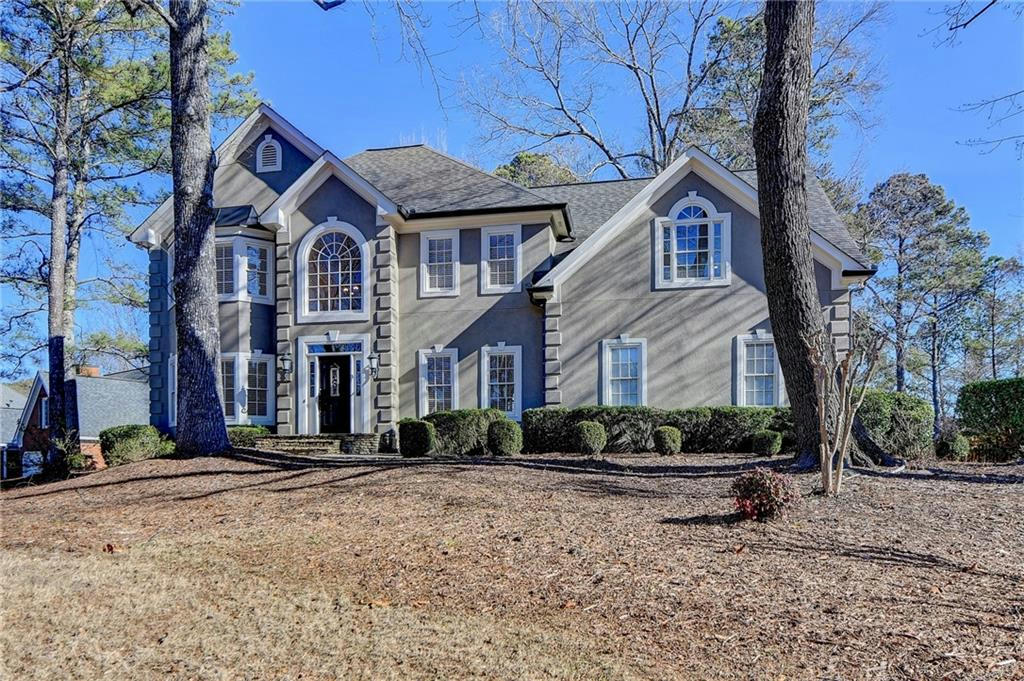The photograph captures a large, two-story, gray house with white-trimmed windows and doors, situated in the upper middle portion of the image. The house features a variety of roof lines and levels, including a rounded front section on the left, a prominent doorway to the right of that, followed by a flat wall with four windows, and another section further right with its own peaked roof. This rightmost section includes a window on the top floor and two on the bottom floor. 

In front of the house runs a row of green hedges extending from the right of the door along to the end of the house. The foreground, particularly the lower part of the image, is dominated by a brownish area that appears to be dead grass, with a hint of leaves scattered, giving a sandy appearance closer to the house. Further back, the yard transitions into a lighter tone at the bottom left corner. 

Several large trees are also present in the scene. A big tree stands slightly to the left of the doorway, its branches and leaves extending upwards and out of the image. Another large tree is visible in the distance behind this one. On the right side of the house, another tree trunk is seen in the foreground, its branches also disappearing out of the frame. 

Behind the house and to the right, additional trees can be seen, blending into the bright blue sky that spans the background without a cloud in sight. Amidst this greenery, a small, seemingly alive bush is visible towards the right side near the brown grassy area.